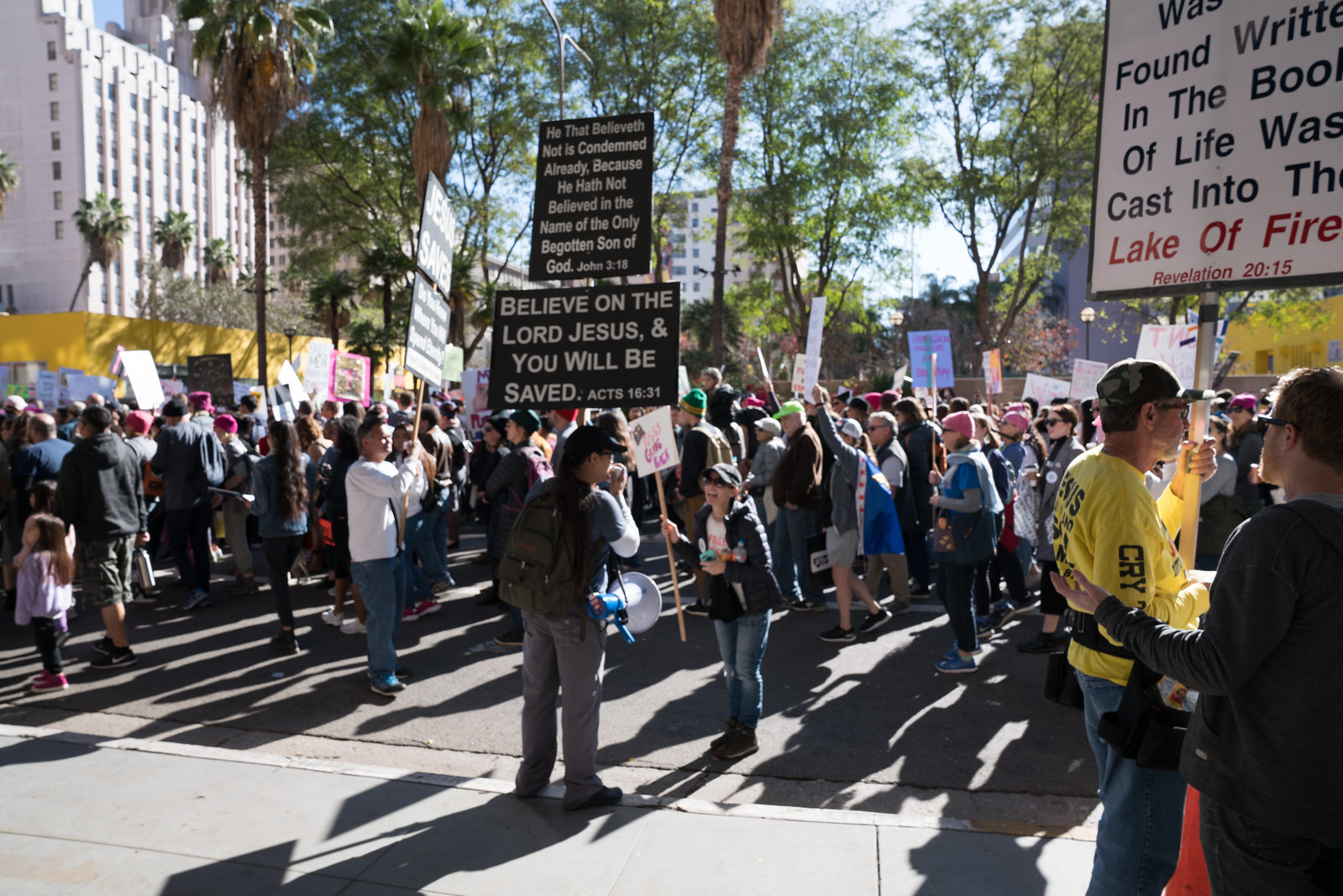In this full-color daytime photograph, a large group of people is engaged in a Christian protest in a metropolitan area. The scene is bustling with many men, women, and children holding up signs attached to wooden sticks, though most of the messages are difficult to read. One prominent sign in the middle of the image stands out with a black background and white text, which reads, "He that believeth not is condemned already because he hath not believed in the name of the only begotten Son of God. Believe on the Lord Jesus and you will be saved. Acts 16:31." Another partially readable sign references being "cast into the lake of fire." The protesters, clad in jackets and long sleeves, suggest a brisk day. Some of them walk along a concrete sidewalk while others are on the street, and one person at the front holds a megaphone and a sign prominently displaying, "Believe on the Lord Jesus and you will be saved." The background features a bright blue sky, sunlight streaming through tall green trees and palm trees, and several towering white buildings with many windows.